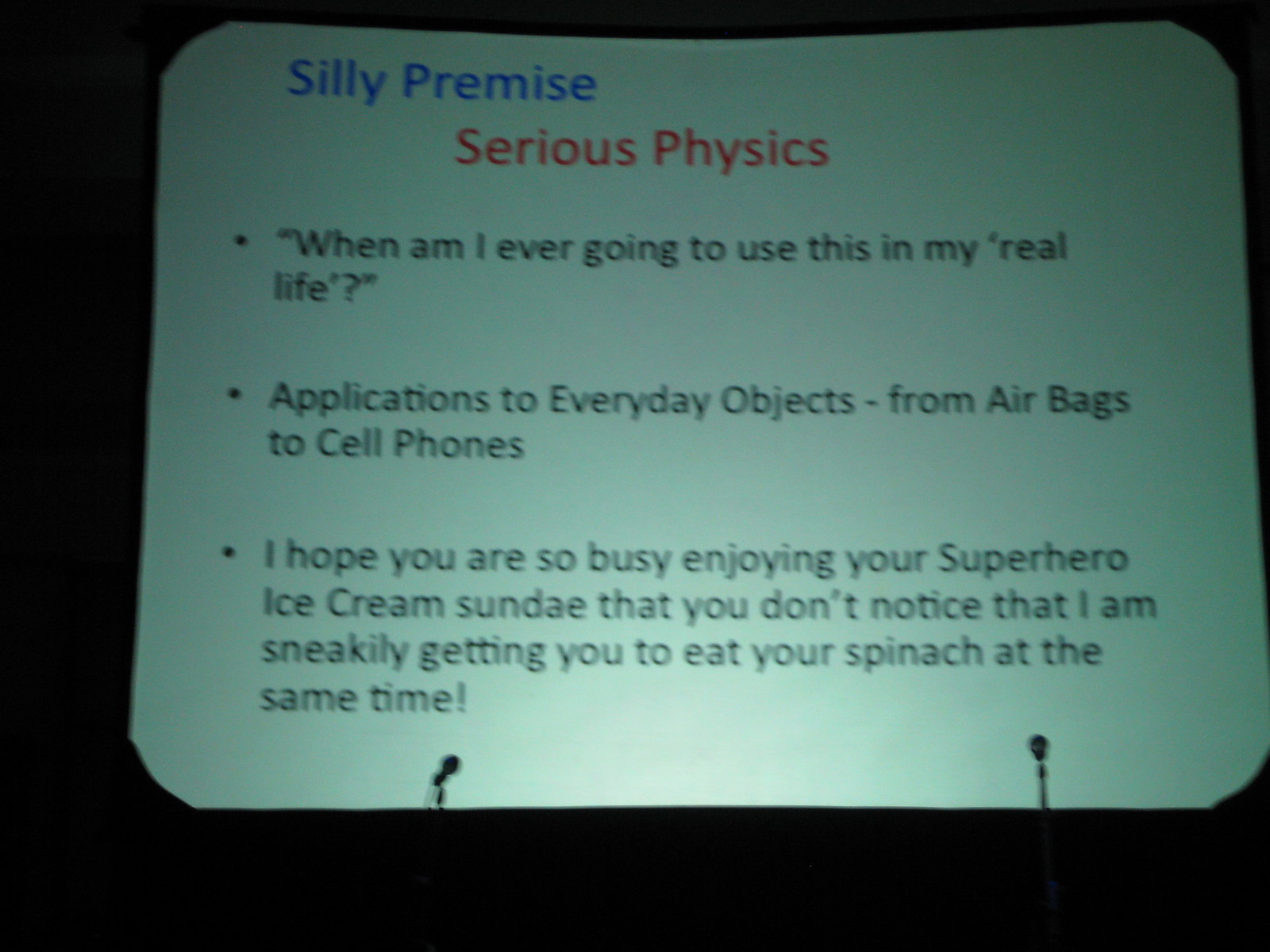The image depicts a photograph of a slide projected on a screen against a black background. The slide features a green square with curved corners, prominently displaying the title "Silly Premise" in blue text at the top. Below the title, "Serious Physics" is written in red. There are three bullet points on the slide:

1. "When am I ever going to use this in my real life?"
2. "Applications to everyday objects - from airbags to cell phones."
3. "I hope you are so busy enjoying your superhero ice cream sundae that you don't notice that I am sneakily getting you to eat your spinach at the same time."

At the very bottom of the green square, there are two tiny black microphones. The overall lighting is dim, suggesting this is a projected presentation rather than a printed card or page.